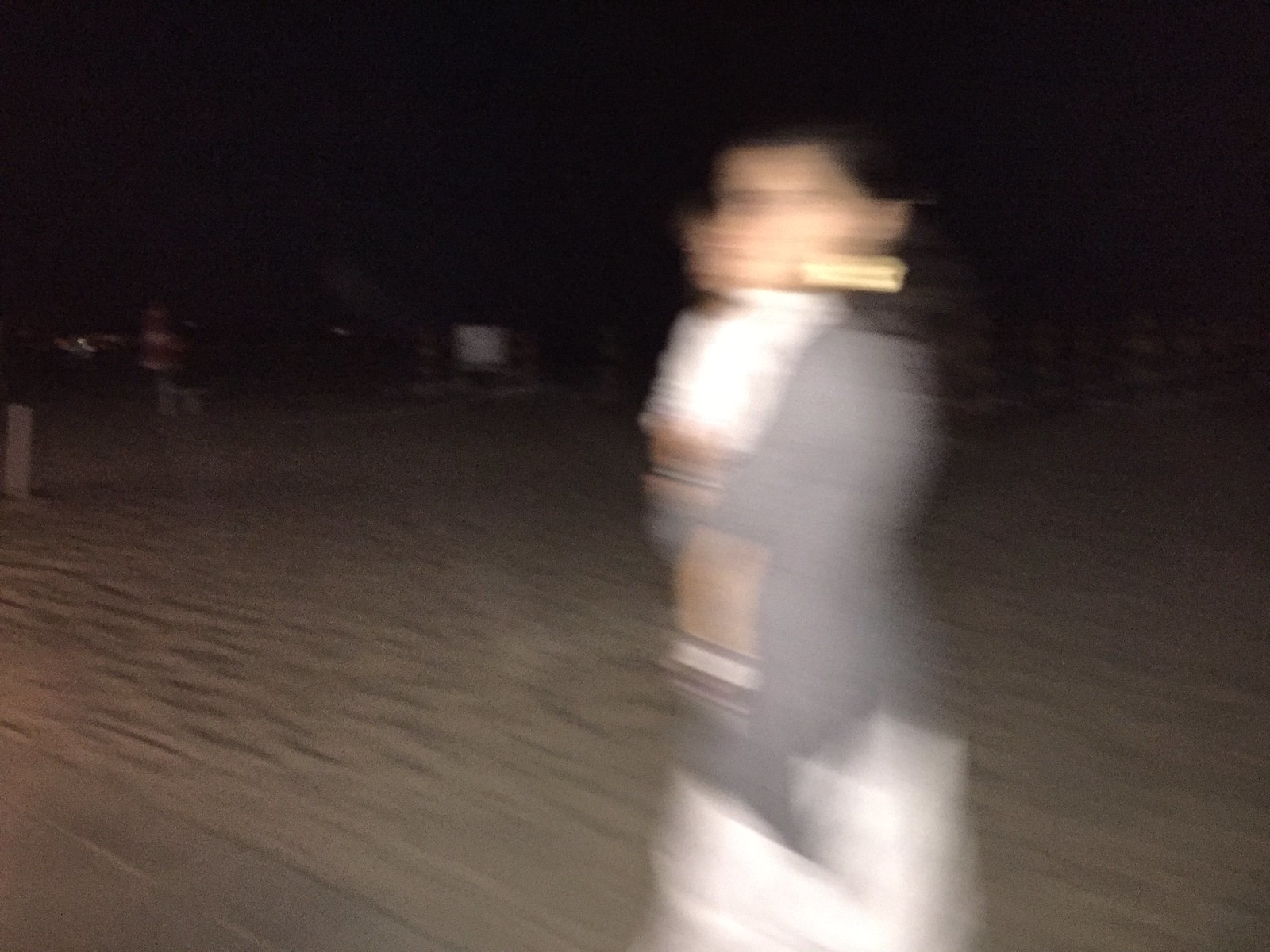This square-shaped image captures a single person standing in the center, although it is extremely blurry and low in resolution, giving an impression of motion. Despite the poor quality, the individual can be vaguely seen wearing a gray top and possibly white pants. Their face is indistinct, making it difficult to discern facial features or any accessories. The ground beneath them has a tan color with a sandy texture, adding to the overall haziness of the photograph.